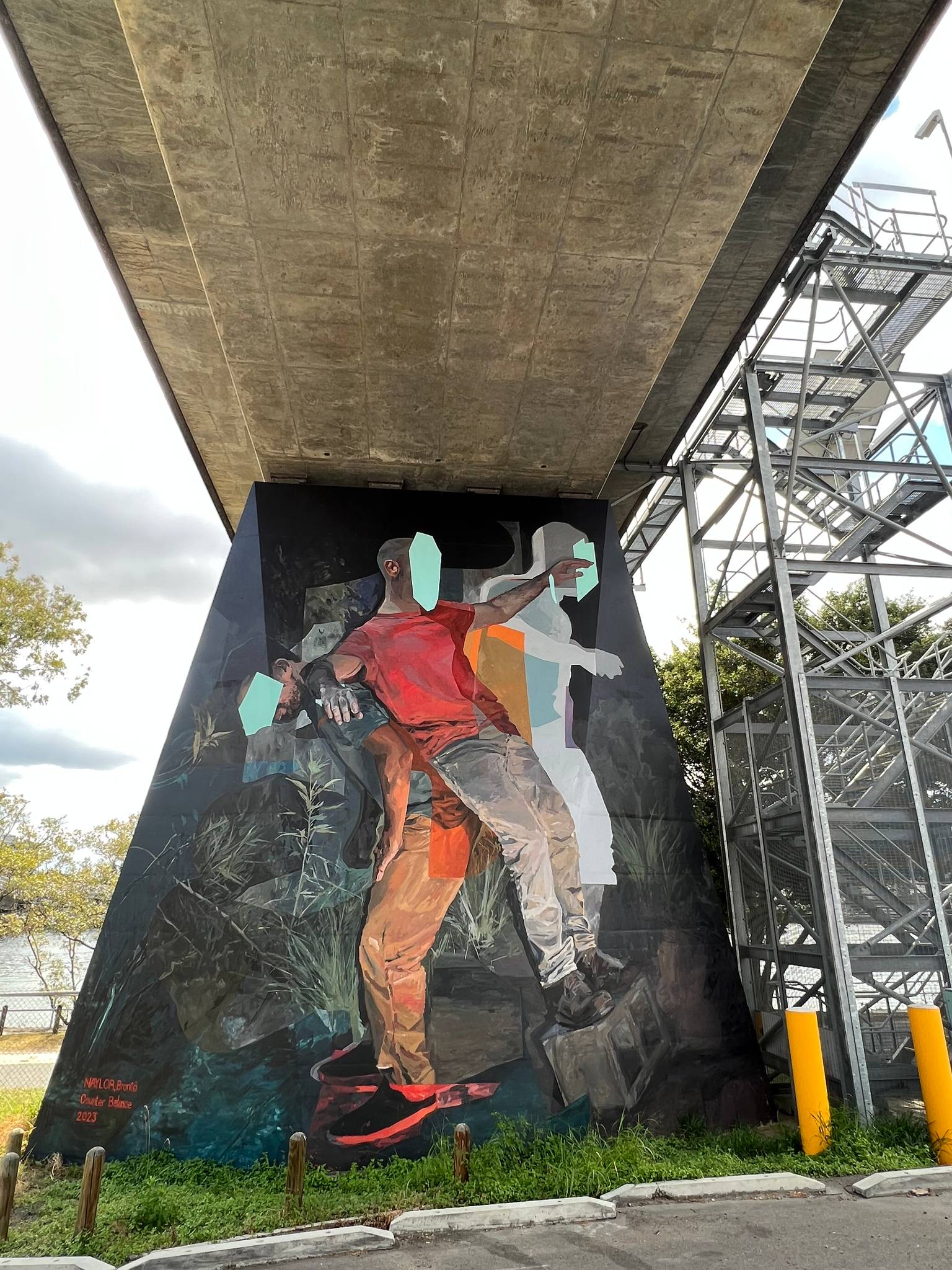The photograph, vertically oriented and full color, captures an outdoor scene under natural daylight. It reveals an urban setting beneath a freeway overpass. The composition foregrounds a vivid piece of graffiti art on a concrete pillar of the bridge, with the overpass's cement underside visible above. The graffiti intricately portrays two male figures; one, wearing a red t-shirt and blue jeans, lies down on his back against another figure clad in a short-sleeved shirt and khaki pants. Both figures' faces are obscured by blue squares. The man on the cinder block, whose arm is raised, sports black shoes, while the other features black and red sneakers. The detailed urban artwork is set against a backdrop of a bright blue sky, trees, and wispy grass. The ground below includes concrete barriers resembling parking stops, and notably, two yellow-painted cement posts stand at the lower right corner. Extending upward from the ground, a silver metal staircase zigzags several stories high on the right, adding an industrial element to this meticulously detailed urban scene.